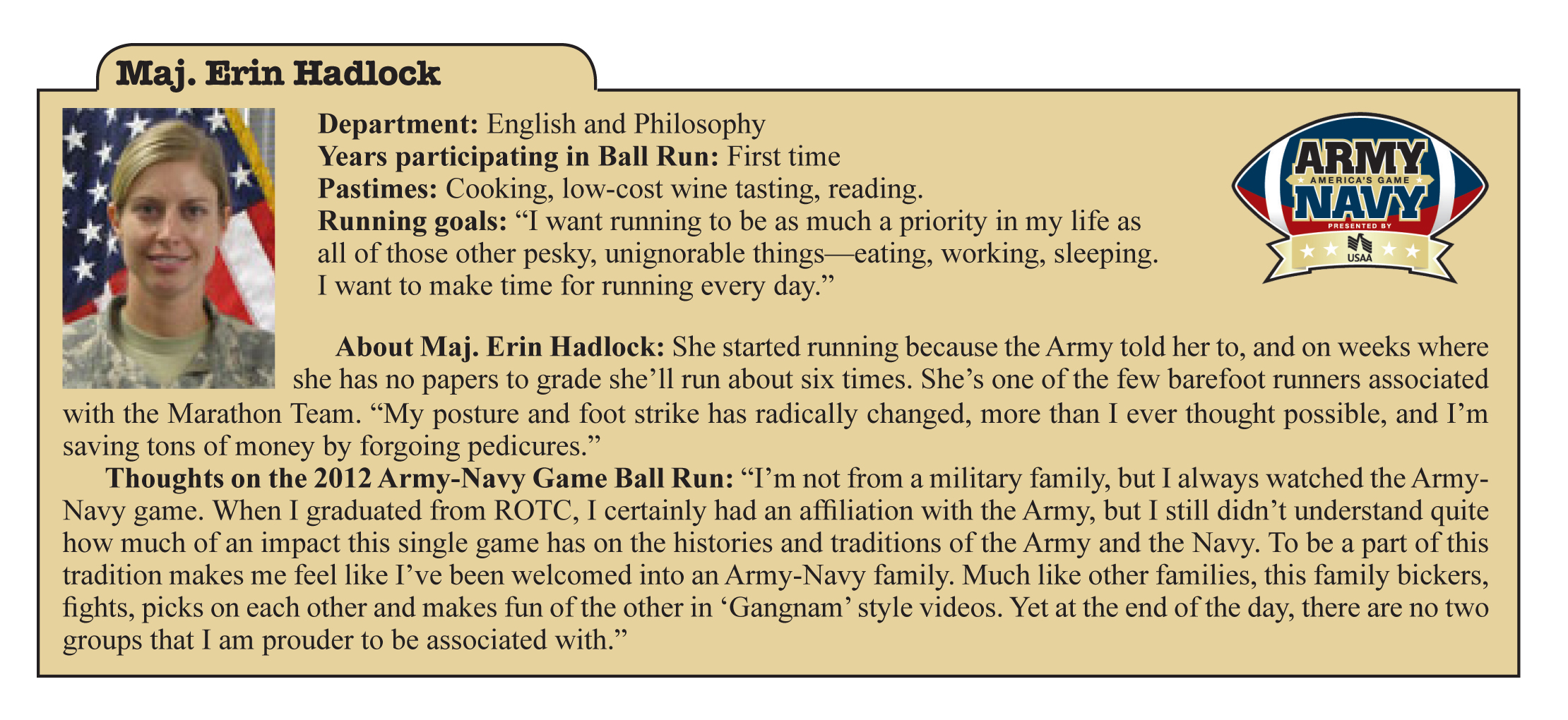The image resembles a detailed note card featuring a profile of Major Erin Hadlock. Positioned in a beige square bubble at the very top-left, the biography introduces Major Hadlock with bold, black dot text. A picture of her in military fatigues, showing her blonde hair with the United States flag in the background, accompanies the text. 

It states her name, "Major Erin Hadlock," and highlights her department as "English and Philosophy." This is her first time participating in the ball run. Her hobbies are listed as cooking, low cost wine tasting, and reading. Major Hadlock's running goals are outlined with her desire for running to become as vital as eating, working, and sleeping. She aims to incorporate it daily into her life.

The bio explains that she began running because of the Army and manages to run about six times a week when not grading papers. Additionally, she is noted as one of the few barefoot runners on the marathon team, mentioning that her posture and foot strike have improved significantly and she's saving money on pedicures.

Her reflections on the 2012 Army-Navy game ball run reveal that although she didn't come from a military family, she grew up watching the game and developed an appreciation for the tradition, feeling welcomed into the Army-Navy family. Despite the bickering and teasing within this community, she expresses immense pride in being associated with both the Army and Navy.

In the upper right corner of the image, there is a football labeled "Army Navy-America's Game."